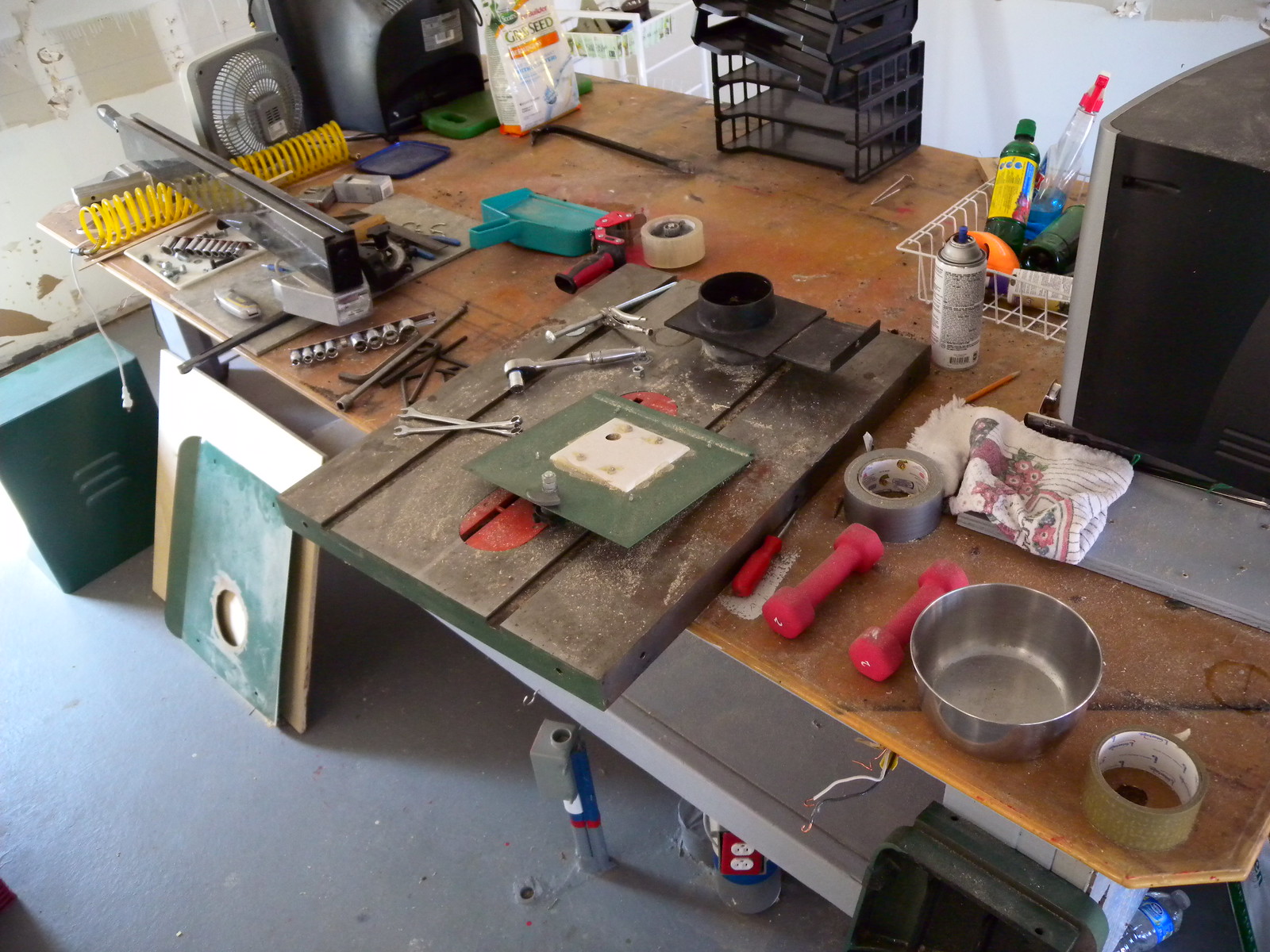A detailed image depicts an assorted collection of tools and materials strewn across a wooden workbench, indicative of an ongoing manual project. The scene is chaotic yet rich with the tools of a tradesperson. Scattered across the table are various components such as hand weights, rolls of tape, screws, metal fragments, and tubing, all coated in a fine layer of dust. Prominently displayed amidst the clutter is a small door, suggesting an assembly or repair in progress, accompanied by nearby mechanical elements likely related to the project. A fan positioned on the table adds to the workspace ambiance, providing much-needed relief or possibly aiding in drying or ventilation. A cloth lies adjacent to the door, hinting at frequent use for cleaning or wiping down surfaces. A spray can is strategically placed, likely for lubrication or painting purposes, and a partially open bag of powder sits nearby, perhaps containing a type of filler or cleaning agent. Also notable are several old televisions awaiting repair, indicating the space serves a dual function for various types of equipment refurbishment. This eclectic assortment suggests a highly versatile and busy work environment dedicated to the restoration and maintenance of diverse mechanical and electronic components.